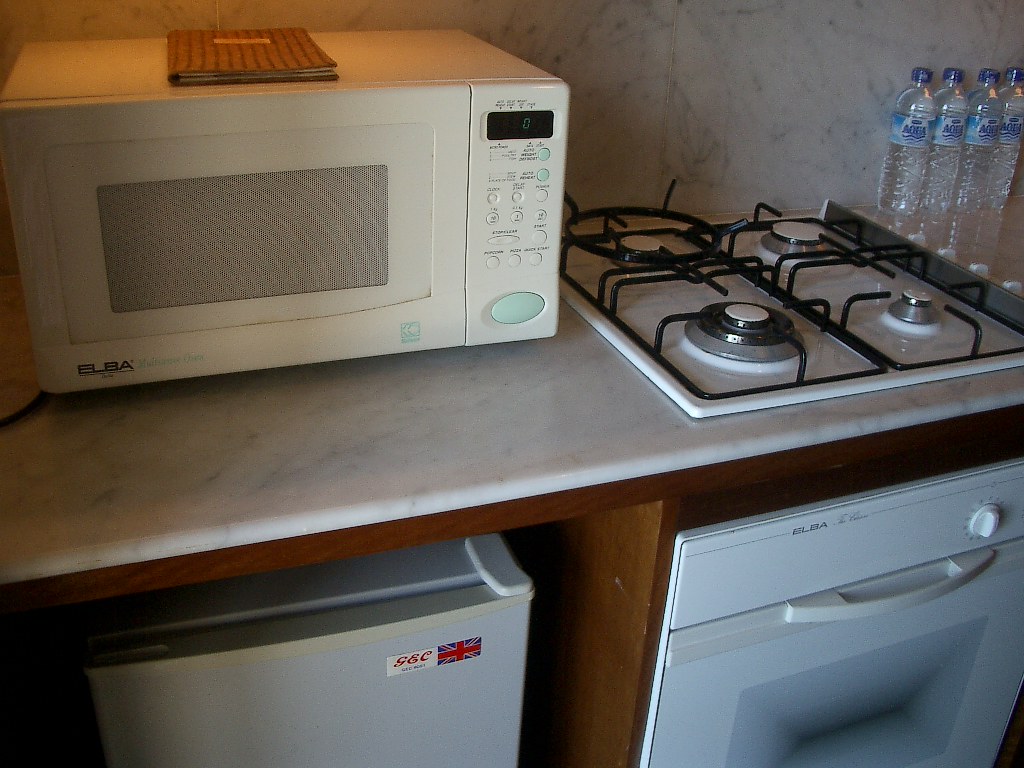This is a color photograph of a compact kitchen area, possibly in a hotel room or studio apartment. The focus is on a white marble countertop with black veining that continues into the backsplash. On the left side of the counter sits a white, digital Elba microwave oven featuring a small screen and buttons, including a notable mint green one on the bottom right. A thin brown book with gold writing, though unreadable, rests neatly on top of the microwave. Illuminating the microwave is a yellow light. Adjacent to it is a white, four-burner gas stove, complete with black grates and a matching white oven beneath it. To the right of the stove, four clear plastic water bottles with dark and light blue labels and caps are aligned against the grey, marbled wall. Below the counter, there is a white mini-fridge on the left, displaying a Union Jack sticker, and a white-handled dishwasher possibly doubling as an oven directly beneath the stove. The overall ambiance suggests an efficiently designed space, with wooden edges around the countertop adding a touch of warmth.